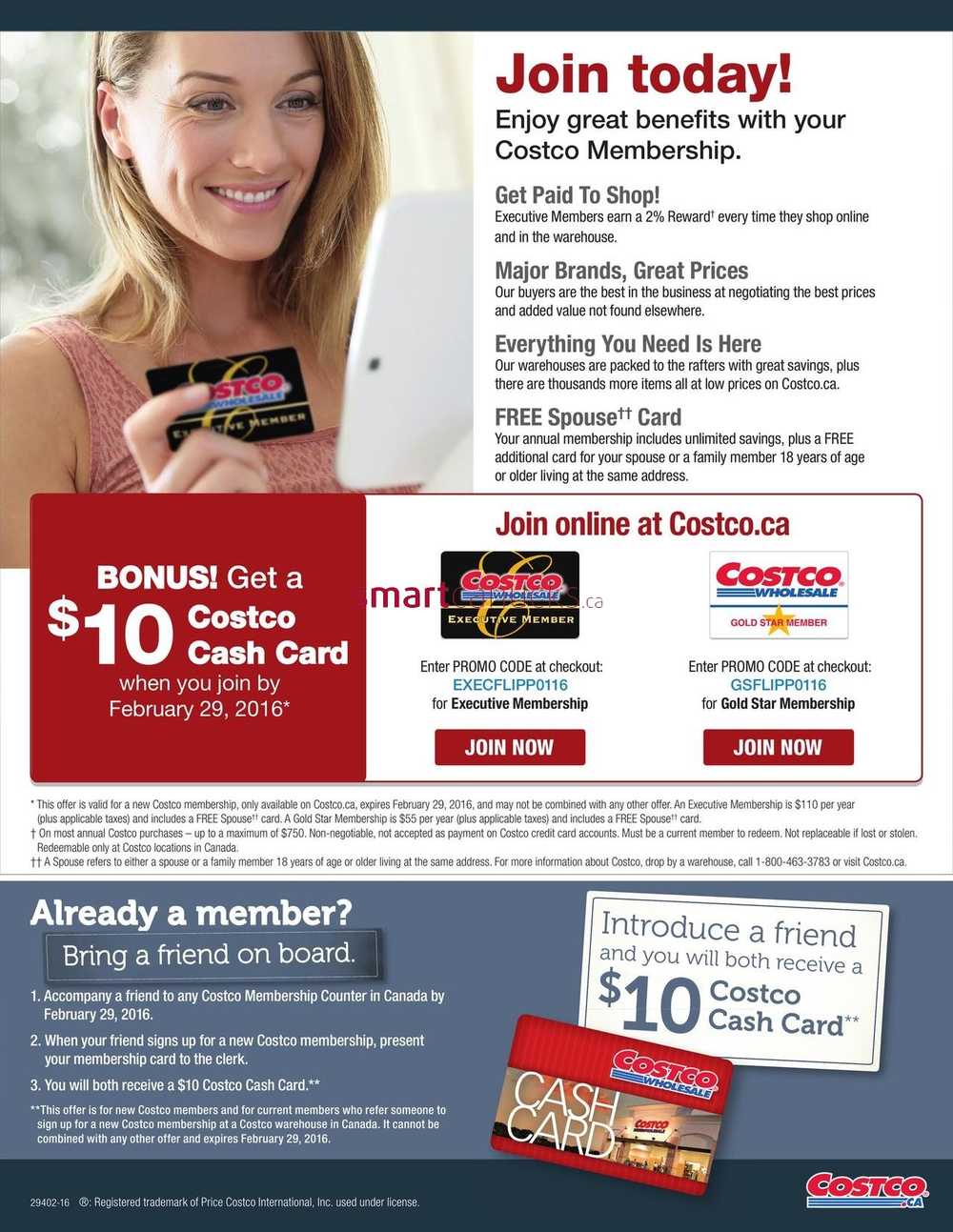The flyer is an advertisement for a Costco membership, prominently showcasing the benefits of joining. To the right, a smiling blonde woman is featured holding up a sleek black Costco Executive Membership card, identifiable by the distinctive cursive "CO" on it. To the left, bold red letters proclaim "JOIN TODAY," with black text underneath enticing potential members with the phrase, "ENJOY GREAT BENEFITS WITH YOUR COSTCO MEMBERSHIP." The flyer emphasizes that an Executive Membership allows members to earn a 2% reward every time they shop, both online and in-store. Detailed descriptions of additional benefits are provided further down.

In the center of the flyer, a rectangle with a red border states that you can join online at costco.ca, indicating the Canadian origin of the flyer. To the right of this, "Costco Executive Membership" is clearly labeled, while to the left, "Costco Wholesale" is mentioned along with information about promo codes available for sign-up. The flyer also details the Gold Star Membership option. Below these sections, the validity of the card and the promotional terms are explained. There is also a note encouraging existing members to refer a friend, located in a darker-shaded section.